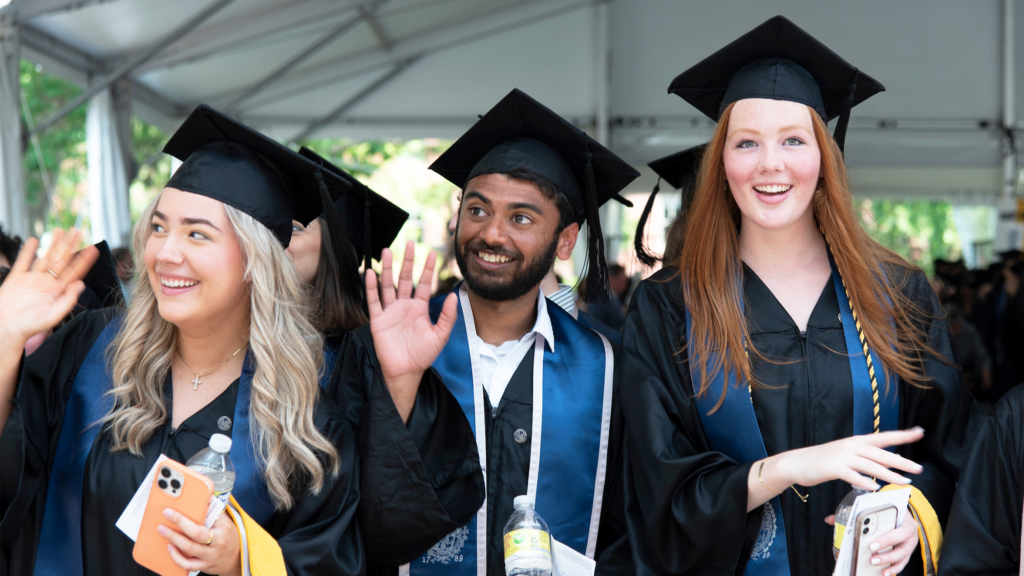In this lively graduation photo, three jubilant college graduates stand together under a large white tent. The background reveals lush green trees with sunlight subtly peeking through, adding a natural aura to the celebration. From left to right, their smiles and gestures speak volumes of their joy and achievement.

On the left, a young blonde woman with white skin is smiling broadly and waving to the right. She’s holding an orange-cased phone and a water bottle in her left hand, embodying the exuberance of the moment. 

In the center, a bearded man of Indian descent also waves, mirroring the woman’s enthusiasm. He’s dressed in a black cap and gown with a vibrant blue sash featuring a white trim. A water bottle rests in his other hand, seamlessly integrating into the shared camaraderie. 

To the right stands a taller red-haired woman with white skin, who smiles warmly while looking slightly upward. She wears a blue sash adorned with a gold cord. In her hand, she holds a phone, a water bottle, and a slip of paper, adding to the cohesive visual theme.

All three are clad in traditional black graduation gowns and caps with blue ribbons cascading down, indicating their academic accomplishment. Blurred figures of other students and a barely visible arm add depth to the scene, hinting at the broader celebratory environment surrounding them.